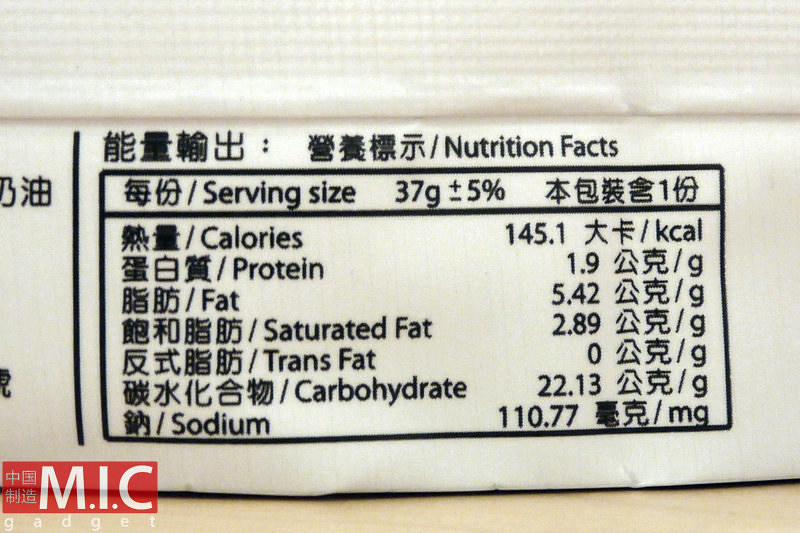This image is a close-up of a nutrition label featuring a rectangular layout and adorned with Asian characters, denoting its origin as an Asian product. The label does include several details in English: 

- The serving size is specified as 37 grams, with a tolerance of plus or minus 5%.
- The calorie content is listed as 145.1 KCal.
- The protein content is marked as 1.9 grams.
- The total fat content is 5.42 grams, with saturated fat making up 2.89 grams and explicitly stating that there are no trans fats.
- The carbohydrate content is detailed as 22.13 grams.
- The sodium level is noted to be 110.77 milligrams.

The information is meticulously presented, providing a comprehensive nutritional profile of the product.